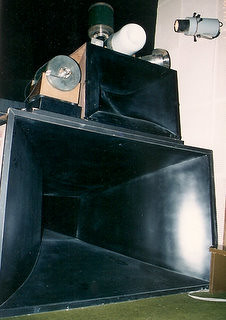This indoor photograph, although low resolution and somewhat pixelated, clearly showcases a pair of vintage-style loudspeakers with an open, concave design. The speakers are positioned one on top of the other on a green carpet. The larger, oversized speaker at the bottom features a matte black front that curves inward towards a smaller square opening. Its wooden body adds a classic touch to its design. Sitting atop the larger speaker is a smaller speaker that mimics the same build and aesthetics. Both items are unshielded and exposed.

Adjacent to these speakers, several electronic devices can be seen, though their specifics are hard to discern due to the image quality. Among them, a particularly noticeable item appears to be a silver disc fixed onto a rectangular black platform, with an array of wires trailing behind it. Additional mechanical components, canisters, and possibly a lightbulb are scattered around, adding to the intricacy of the scene. Mounted on the top right corner of the wall is a device with a circular end, which might be a microphone or a video camera.